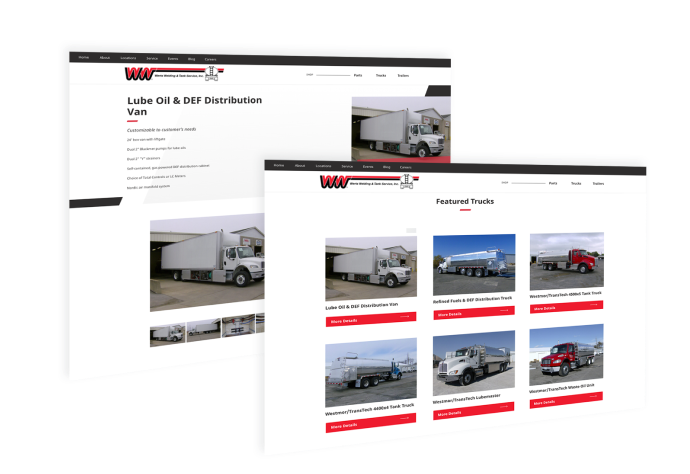The image presents a detailed computer interface with a 3D perspective tilted to the side, showcasing an array of options and images. A prominent black line runs horizontally at the top of the screen. Below it, the text "WW" appears, followed by a lengthy red line. Directly underneath, the "WW" is highlighted with a black area beneath and another black line extending to the side.

On the right, there is an image of a white semi-truck backed into a building. To the left, black text reads "Lube Oil and DEF Distribution Van," underlined in red. Below this, seven small, illegible text options are displayed vertically. The white semi-truck image reappears, backed into a building, mirroring the previous depiction.

Further to the right, another computer screen is shown with a similar 3D effect. It features a title, "Featured Trucks," above multiple rows of vehicle images. Each row displays different models:

1. The first row includes:
   - A white semi-truck.
   - A truck with a silver cylindrical back.
   - A red and white truck.

2. The second row features:
   - Another white semi-truck.
   - A white truck with a long silver cylinder attached to the back.
   - A red semi-truck.

The detailed interface highlights the versatility and options available for various truck models in a sleek, visually engaging manner.